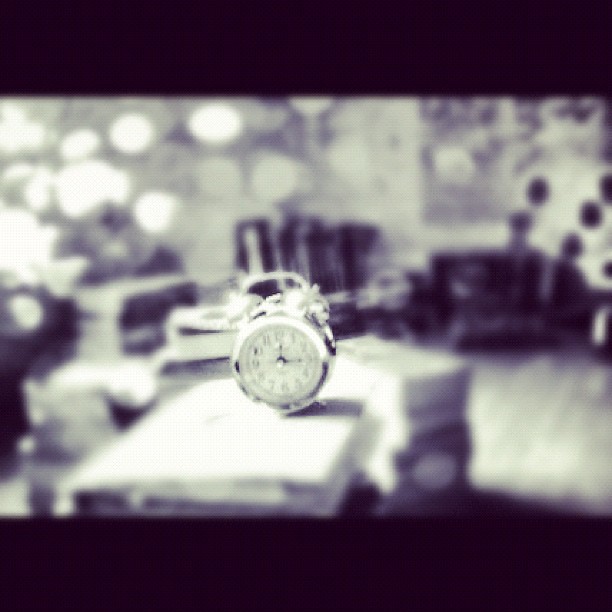A captivating black and white photograph showcases a vintage-style round clock with a pair of bells perched on top, resting serenely on a stack of books. Despite the monochrome palette, the clock's silver hue subtly gleams, enhanced by the light reflecting off its polished surface. The photograph features deliberately out-of-focus background, highlighting the clock's intricate details. The clock face clearly displays the time as 12:15, surrounded by evenly spaced numerals. Above the clock face, a small silver handle can be seen nestled between the twin bells. The composition is framed with black borders both at the top and bottom, adding to its classic charm. Additionally, the top left corner of the image is adorned with a series of light reflections, resembling small round orbs, enhancing the overall visual appeal.